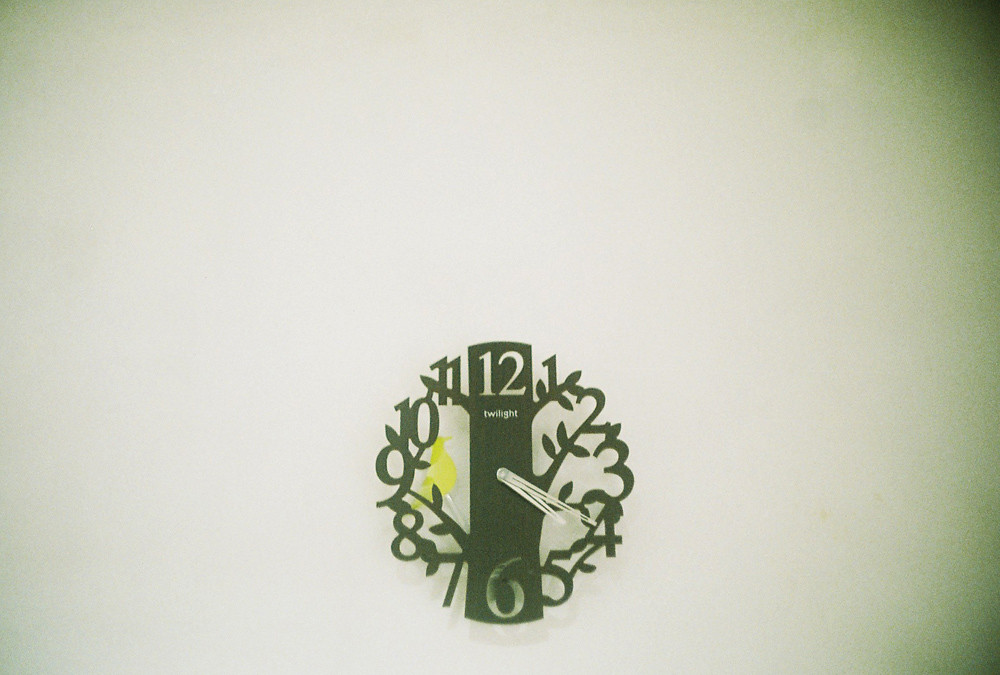In this visually captivating image, we are presented with a landscape-style photograph featuring a decorative clock as the main focal point. The backdrop is predominantly white, transitioning into a dark black gradient at the corners. The clock, which is circular and appears to be meticulously drawn on a piece of paper, embodies an exquisite blend of nature and time. Intricately crafted, the clock's center is formed by a tree trunk, with branches extending outward, seamlessly integrating the numbers 1 through 12, resembling leaves in a clockwise arrangement. These elements are rendered in a subtle greyish-brown hue, giving it an artistic and organic feel. Notably, there is a yellow bird perched near the 9 o'clock position, adding a touch of vibrancy to the monochromatic scheme. The clock's hands, indicating the time 4:20, are white, standing out against the tree-themed design. At the 12 o'clock mark, the word "twilight" is inscribed, blending into the naturalistic motif. This image is a masterful interplay of shadows and light, with dark gradients around the corners, creating an ethereal and immersive visual experience.